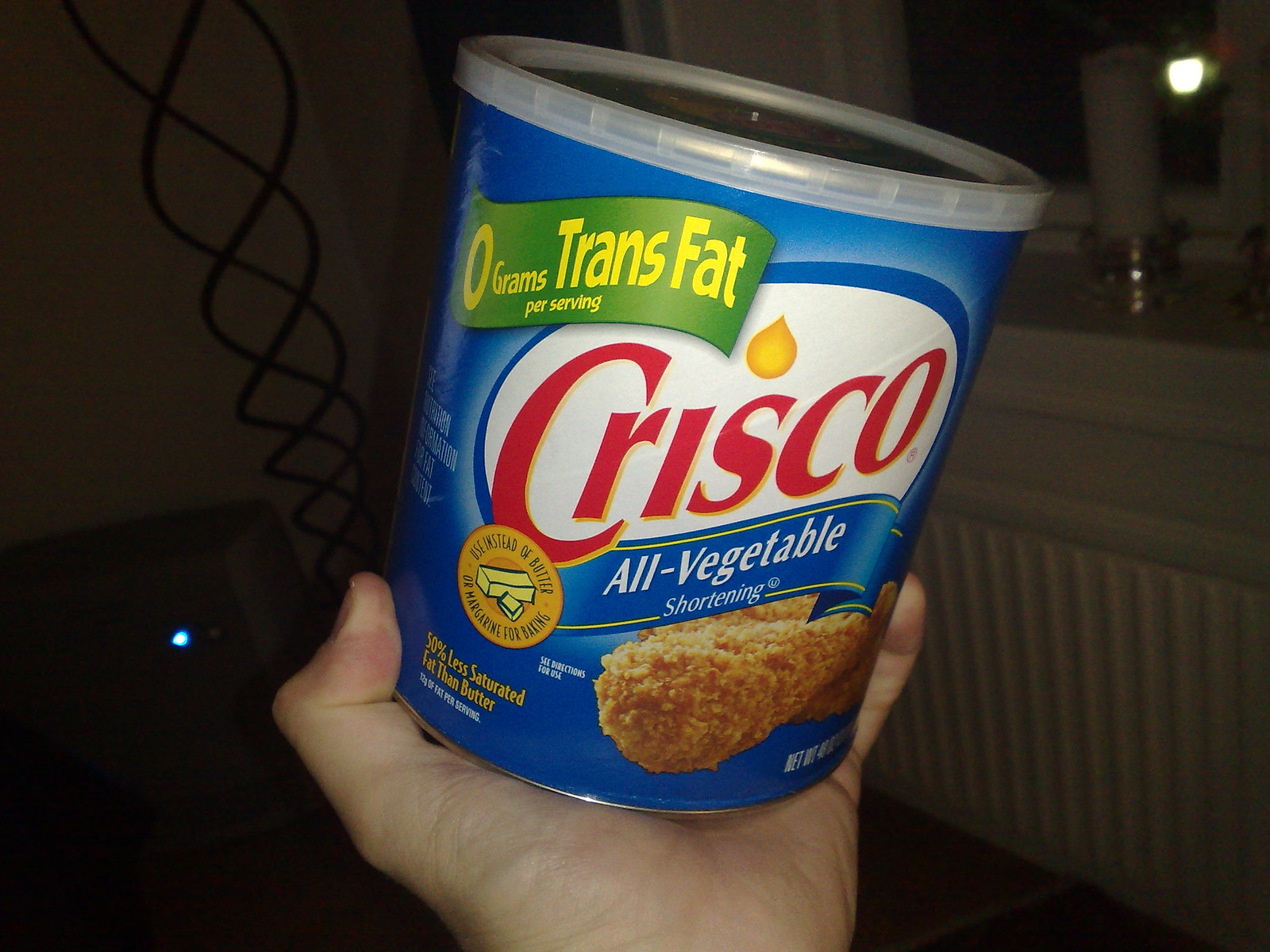A hand is outstretched, holding a cylindrical container. At the top, it features a plastic lid. The main body of the container is blue, adorned with a green ribbon on the top left. Prominently, the front displays a white circle with a blue rim, containing bold, red lettering spelling "Crisco." Above the text, there is a flame symbol over the "S". Below "Crisco," a blue ribbon with white text indicates "All-Vegetable Shortening." To the left of this is an orange circle depicting a stick and square of butter. The very bottom of the container showcases an image of golden, breaded fried chicken with a large pickle. The lower left corner states "50% less saturated fat than butter." There is some light shining on the right side of the container, obscuring additional details. The container advertises "zero grams trans fat per serving."